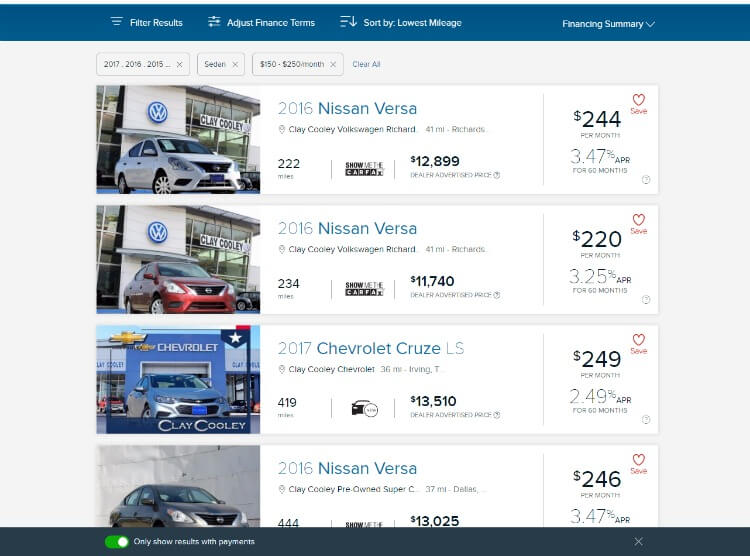Caption: 

The image displays a web page from a car listing site with various search and filtering options. At the top, a blue navigation bar allows users to filter results, adjust finance terms, and sort the listings by criteria such as the lowest mileage. To the right, there’s a financing summary, with sorting options by year, namely 2017, 2016, and 2015, and a category filter set to "Sedans." Users can clear all filters if needed. 

The search results show four cars:

1. A 2016 Nissan Versa with a monthly payment of $244.
2. Another 2016 Nissan Versa priced at $220 per month.
3. A 2017 Chevrolet Cruze LS with a monthly payment of $249.
4. A third 2016 Nissan Versa valued at $246 per month.

The billing range indicated is $150 to $250 per month.